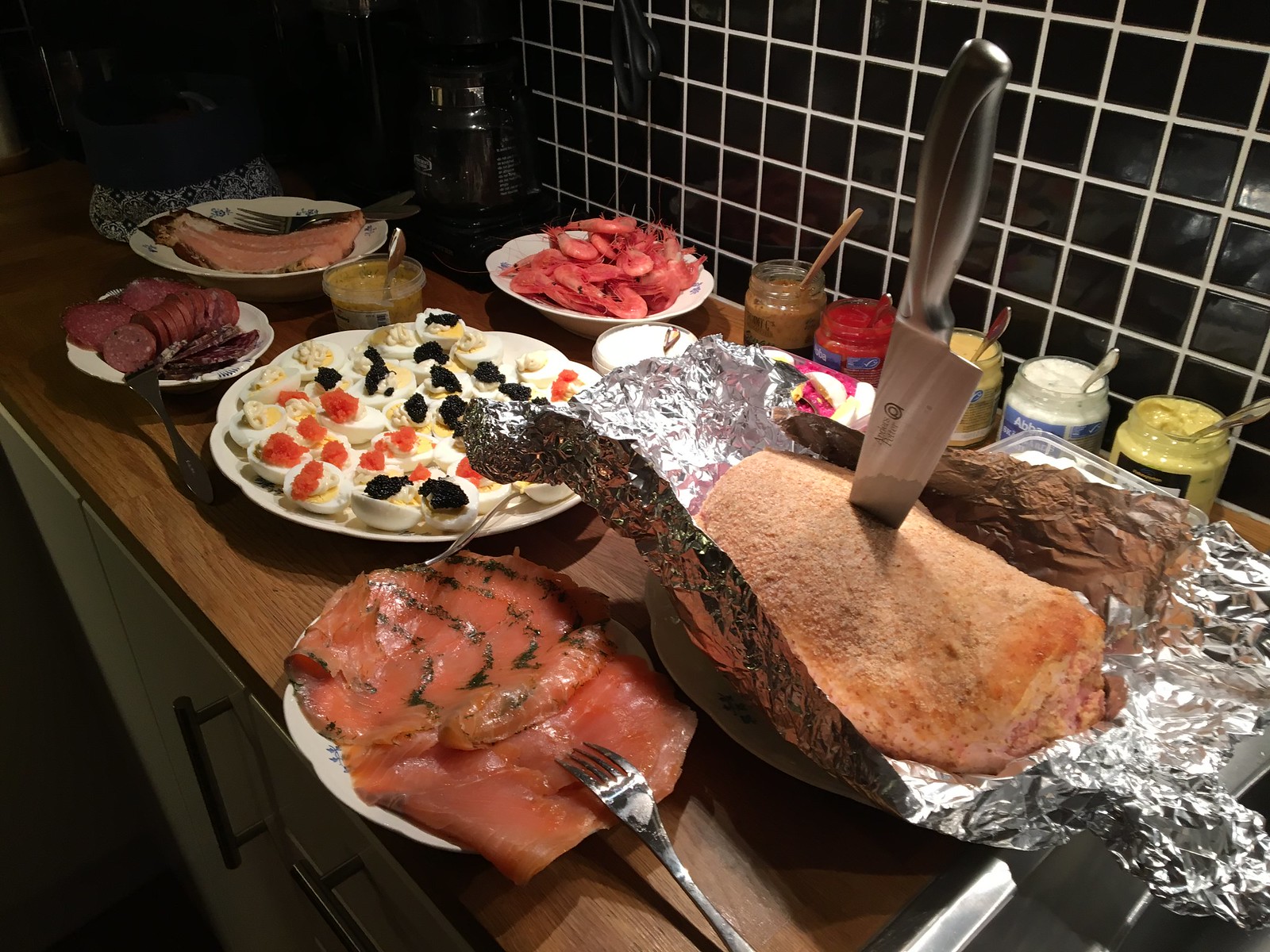This image captures an abundant meal spread meticulously laid out on a wooden kitchen counter, framed by a striking black and white checkered tile backsplash. In the foreground, a plate of smoked salmon with a fork rests invitingly. Close by, a large ham, ceremoniously unwrapped from tinfoil, has a knife embedded in it, centered on another plate. Arrayed behind the ham are five distinct jars of condiments, likely mustard, mayonnaise, ketchup, and possibly Worcestershire or barbecue sauce, showcased in yellow, white, red, and brown hues. A bowl of pink prawns gleams beside a platter of deviled eggs, intriguingly adorned with red and black caviar. Further back, a plate of sliced sausages and another one featuring filleted mackerel complete the assortment. All the dishes are presented on pristine white plates, enhancing the visual appeal of this culinary display. The scene suggests an indoor kitchen environment, and the photo, taken from an overhead angle, beautifully captures the diverse colors and textures of this elaborate feast.